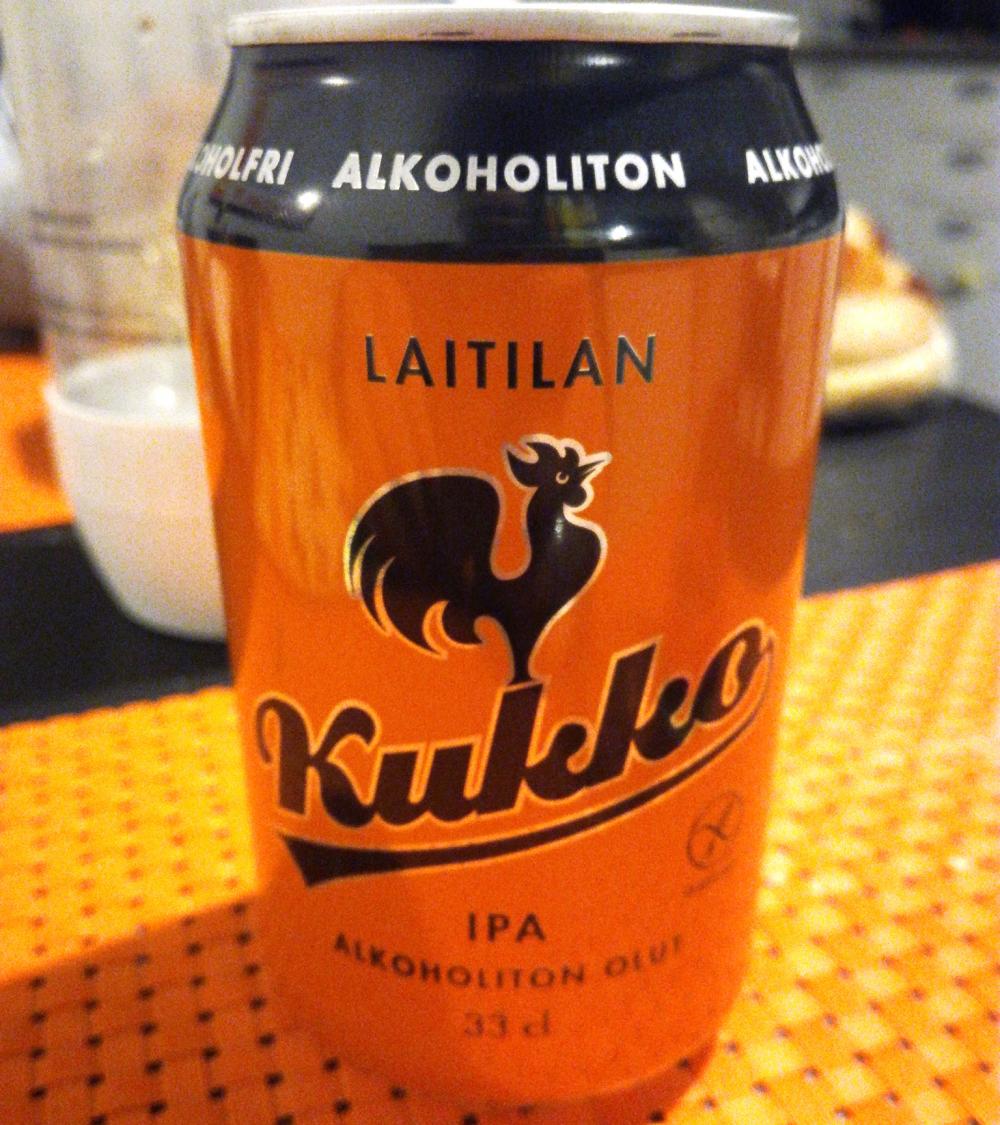The image features a close-up color photograph of an orange metallic beverage can with a shiny surface, positioned on what appears to be a kitchen table or counter with other tableware in the background. The can has a distinctive black ring around its top with capitalized white letters spelling “A-L-K-O-H-O-L-I-T-O-N.” Below this, the main label showcases black writing on an orange background. At the top of the label, the word “L-A-I-T-I-L-A-N” is prominently displayed. Central to the design is a detailed drawing of a rooster standing and facing to the right, which emanates from the top of the letter ‘K’ in the word “K-U-K-K-O,” written in a flowing, angled script beneath the rooster. Below this, “IPA” is clearly marked along with the volume and alcohol measurements, further highlighting the product as an alcohol beverage. The image also includes the repeated word “Alcoholiton” and additional text potentially reading “O-L-U-F 33cl,” along with a secondary X-in-circle icon situated to the right of the logo.